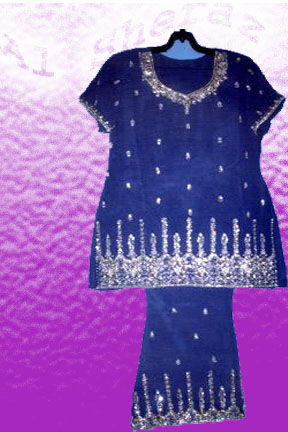Set against a textured purple background that transitions from a light pinkish-purple at the bottom to white at the top, the image prominently displays "A1, Shiraz" in text curving along the upper portion. Central to the image is a hanger holding a dark blue skirt suit adorned with intricate silver beadwork. The top features short sleeves trimmed with silver, a collar edged in silver, and a hem decorated with alternating long and short silver lines, reminiscent of the points on a crown. Vertical lines of silver dots run down the top's bodice. The matching skirt, half the width of the top, also flaunts silver dots—sporadically dispersed—and a hem with a similar alternating pattern of long and short silver decorative lines. The overall design evokes elegance and attention to detail, suggesting its use in a clothing advertisement.